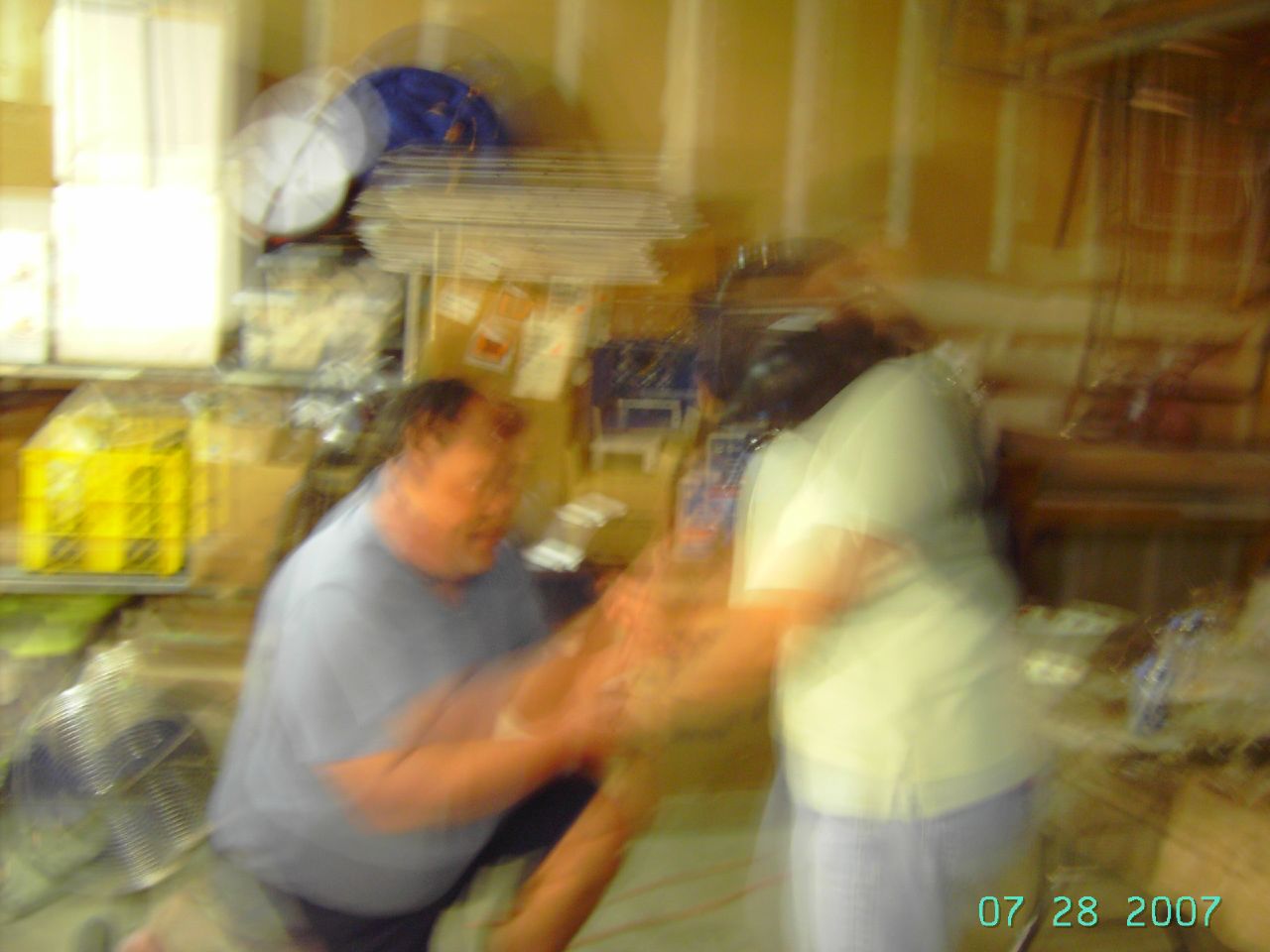In this rectangular, extremely blurred photograph, the setting appears to be within a warehouse or garage characterized by unfinished walls. Two men are centrally featured: the man on the left is overweight, wearing a gray t-shirt, and is grasping the other man, who is dressed in a yellow t-shirt and gray sweatpants or pants. Both men are looking toward each other. In the lower right corner, a timestamp in light green digitally displays "07 28 2007." Behind them, yellow milk crates are stacked on a shelf affixed to the wall, alongside a metal scale located near an open window in the upper left corner. The floor remains indiscernible, but the walls are constructed from light-colored wood.